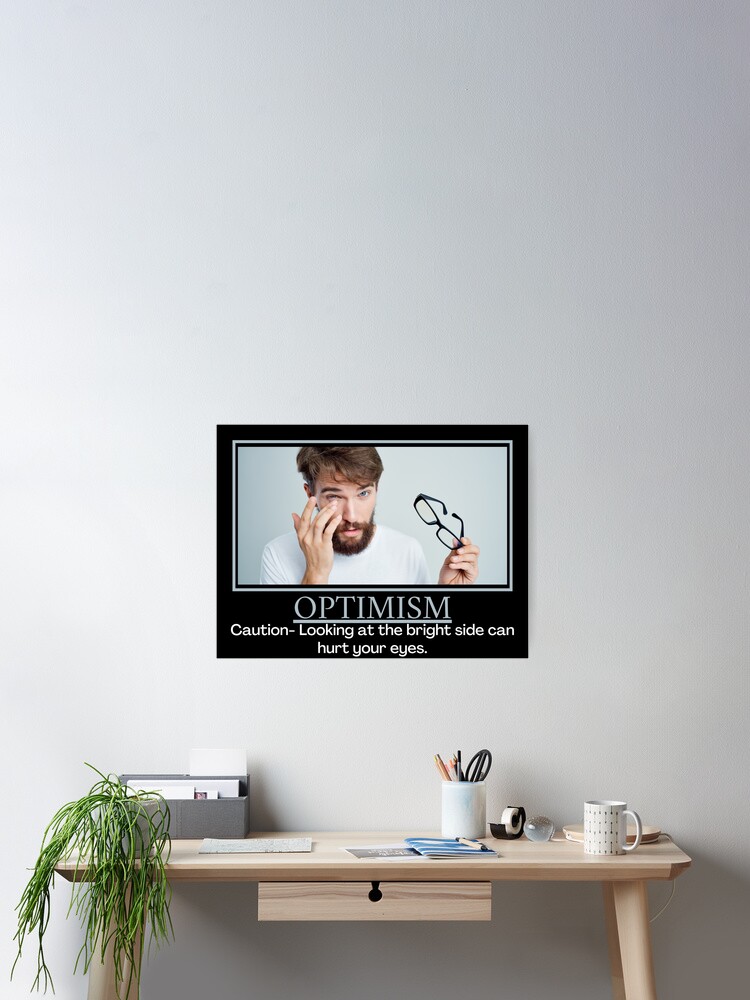This is an image of a minimalistic desk set against a completely white wall, featuring a light-colored wooden surface with four legs. The desk includes a middle drawer, which appears to have either a keyhole or handle, though it's not clearly distinguishable. On the desk, several items are neatly arranged: a wilting green plant is situated at the bottom left corner, while a white coffee mug is at the bottom right. A white lamp is placed at the top right corner. Along the back edge of the desk are an organizer for paperwork or books, a small keyboard, a collection of books in the bottom middle section, a pen holder with pencils and black scissors, and a tape dispenser at the top right. Above the desk, there is a black-framed poster featuring a man with brown hair and a beard, wearing a white shirt and rubbing his right eye while holding a pair of glasses in his left hand. The poster reads: "Optimism, Caution, looking at the bright side can hurt your eyes."